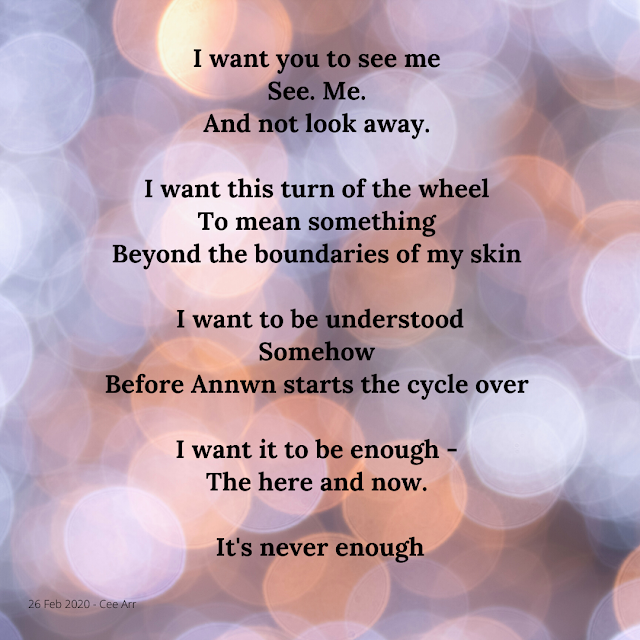The image features an inspirational poem written in bold black text against a background of softly hued neutral shades of grey, purple, pink, and white. The background consists of overlapping circle shapes which resemble a mix of blurred spots of light or delicate bubbles underwater. These circles vary in color, ranging from soft whites and greys to pale blues and faint oranges, with some appearing subtly illuminated by a light source. The text reads, "I want you to see me, see me and not look away. I want this turn of the wheel to mean something beyond the boundaries of my skin. I want to be understood somehow, before and when it starts to cycle over. I want it to be enough, but here and now, it's never enough." The overall composition evokes a sense of depth and ethereal beauty, complementing the heartfelt sentiment in the poem.